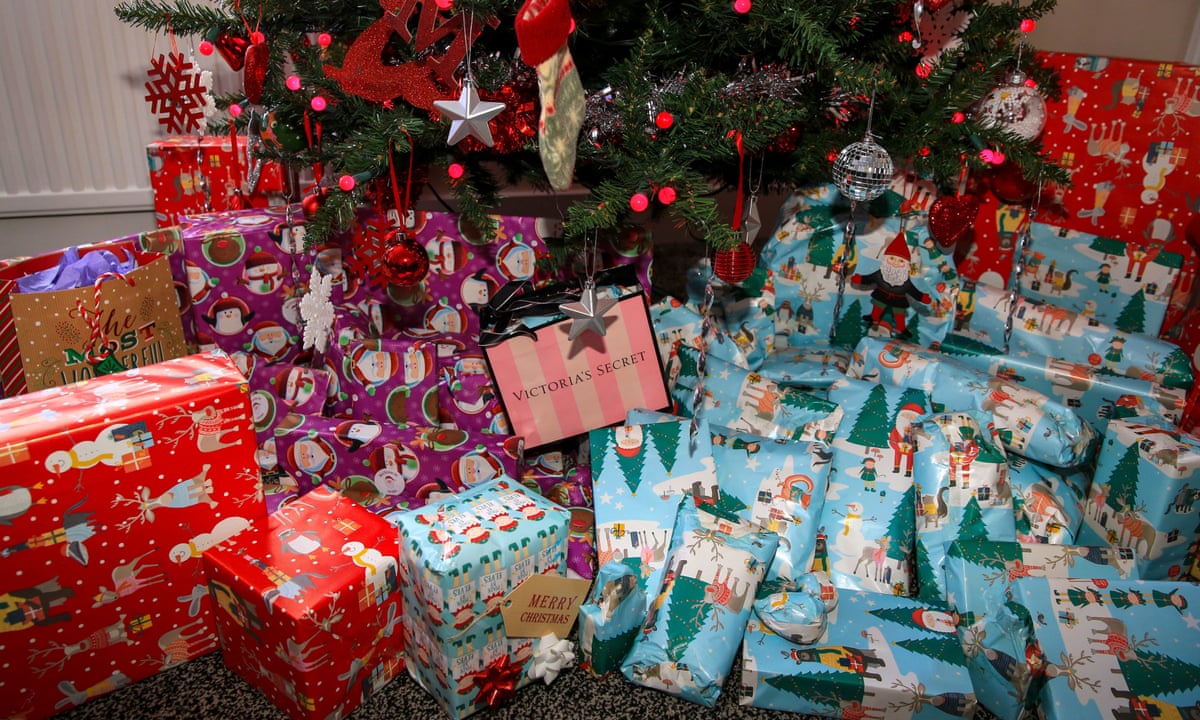This horizontal photograph captures the lower section of a festive Christmas tree adorned with a variety of decorations including a silver star, a miniature disco ball, several red ornaments, traditional holiday ornaments, red snowflakes, a reindeer, and tinsel. The tree, whose green hue suggests a traditional look, stands against a backdrop filled with approximately three dozen gifts of diverse sizes and shapes, wrapped in an array of colorful paper. Predominantly, the presents are cloaked in blue wrapping paper featuring Christmas tree designs, concentrated towards the bottom right of the image. Interspersed among them are gifts wrapped in red and purple paper, the latter adorned with festive motifs such as penguins, snowmen, and Santa Claus. Centrally placed among these gifts is a conspicuous Victoria's Secret bag. This abundant collection of presents, suggesting a gathering for a large family, completely fills the space beneath the gorgeously decorated tree, creating a warm and jubilant Christmas scene.